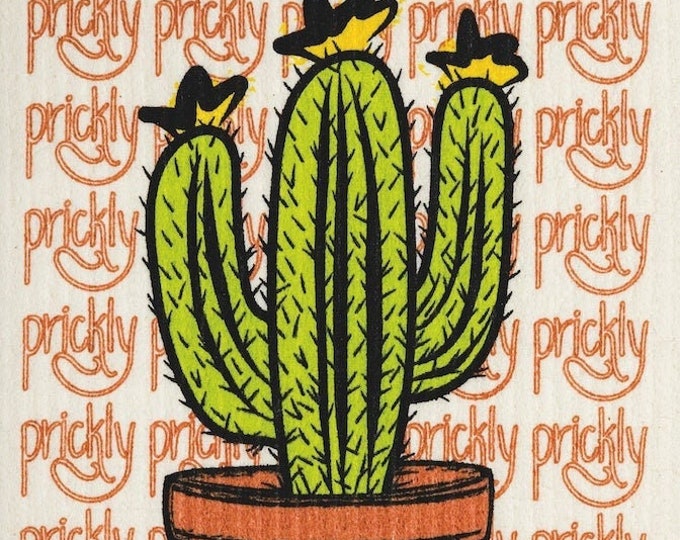The image is a detailed, cartoon-style illustration of a cactus with three prongs, each topped with what appears to be a small yellow hat, reminiscent of a cowboy hat. The cactus is planted in a brown ceramic pot with a black sketched outline, and it features a green body with numerous black dashed lines representing its prickly spines. The background is a pale beige square adorned with a repetitive pattern of the word "prickly" in a clay-colored font, arranged in a 5x5 grid. This stylized text gives the appearance of wallpaper.